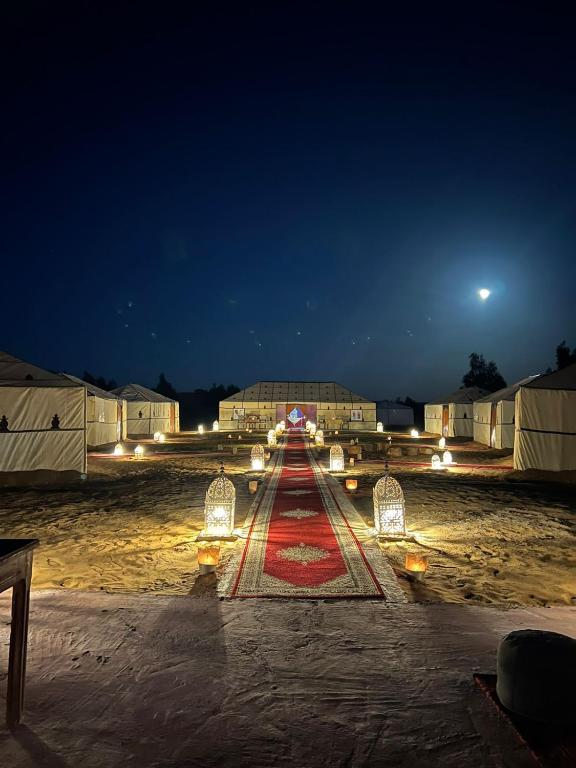The nighttime image depicts a sandy clearing illuminated by the soft light of a full moon positioned in the dark, deep blue sky towards the right-hand corner. The scene features a pathway that divides the clearing, adorned with a red carpet extending from the foreground to a larger ceremonial tent in the background. This red carpet, with hexagonal beige openings in the center, is bordered by gold lines on either side. Illuminating the pathway, a series of lanterns emit a white glow, gracefully lining both sides of the carpet, with additional lanterns situated between the carpet and the tents.

On either side of the pathway are three smaller tents with trapezoid roofs, making a total of six tents flanking the sides, plus the prominent larger tent at the end of the pathway. The area between the pathway and the tents appears to be bare ground or sand. The tiny, window-like openings on the trapezoid-roofed tents contribute to the serene, ceremonial ambiance of the setting, suggesting a campground, religious site, or perhaps a wedding venue. The arched stone structure behind the tents, alongside the carefully arranged lanterns and radiant moon, further enrich the tranquil nighttime scene.